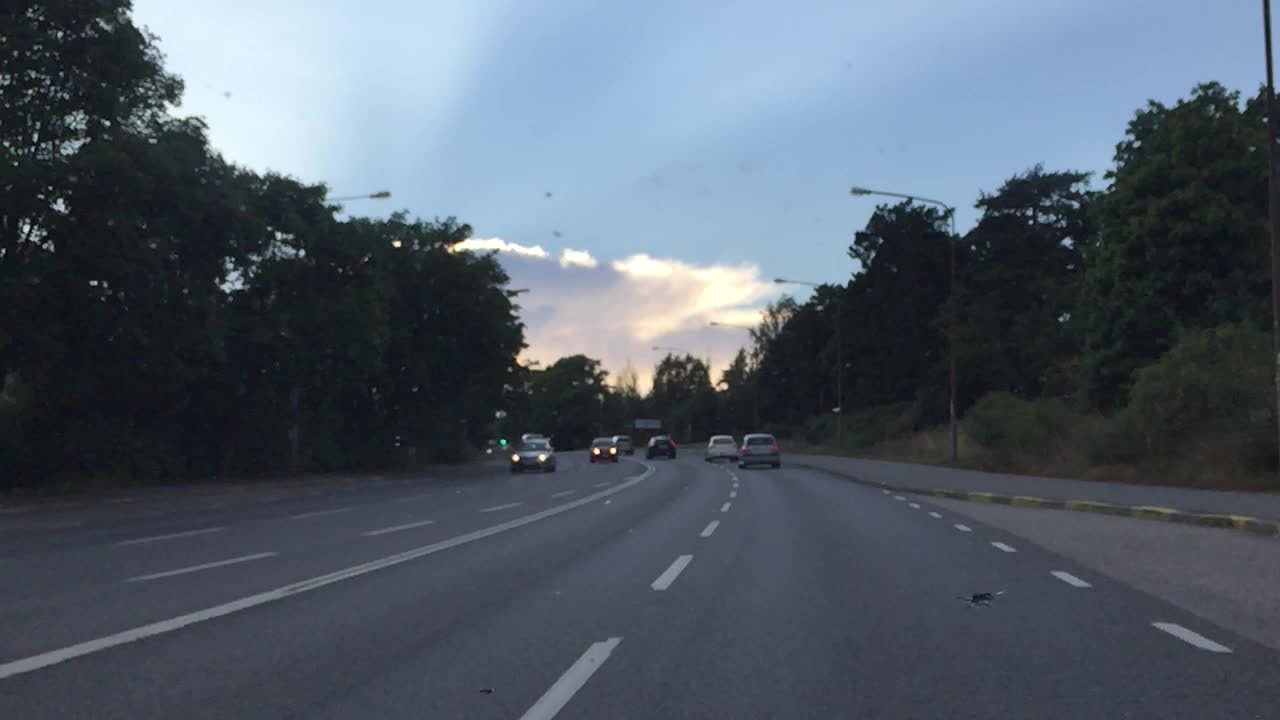This image captures a four-lane, non-divided highway during the twilight hours, curving from the bottom left to the middle and then back to the left of the frame. There are two lanes on each side, with a clear yellow line down the center. On the right-hand side, we observe a white car, a gray car, and a black car, along with several other vehicles, some of which are coming towards the camera with their headlights on. The photograph appears to have been taken from the front of a moving vehicle. The highway is lined with curbs and is flanked by trees on both sides, becoming less detailed as darkness approaches. Several streetlights can be seen along the road, not yet illuminated, adding to the serene atmosphere. In the background, large white clouds with dark undersides display yellow highlights from the setting sun. The sky above transitions from a soft blue to the warmer hues of the sunset, enhanced by thin, wispy clouds. There also seems to be a lane of merging traffic on the left-hand side, contributing to the scene's dynamic flow.